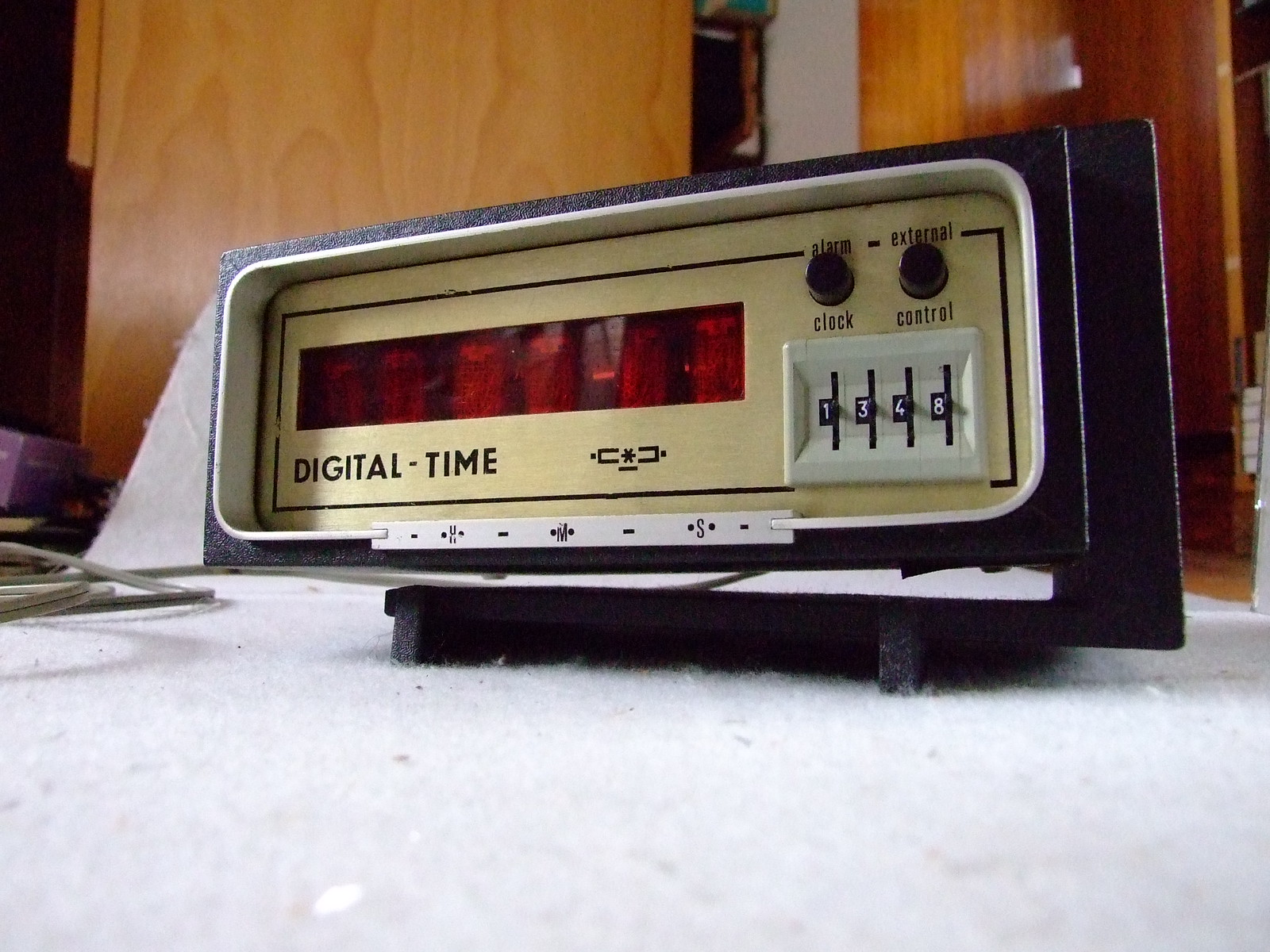A long, rectangular digital clock is perched on a shiny white countertop that appears slightly dusty. The clock, enshrined in a sleek black frame and further accentuated by a larger black plaque behind it, exudes a modern aesthetic. Its gold face, emblazoned with the text "Digital-Time" in bold black letters, complements the red, illuminated digits of the time display. The clock's interface is bordered by another black trim that neatly outlines the inner gold display. Two small, round, black buttons are situated on the clock, labeled "Alarm Clock" and "External Control," respectively.